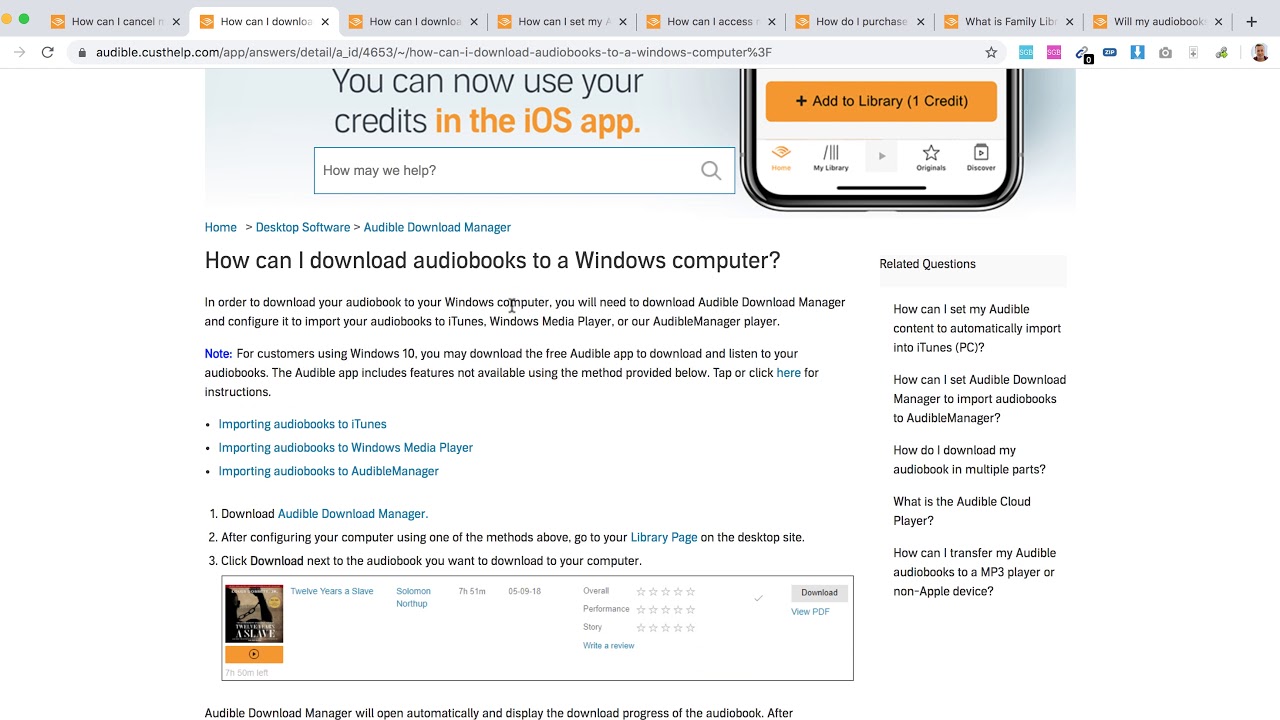This detailed caption accurately portrays the screenshot and its context:

---

The screenshot, captured from a computer screen, displays multiple browser tabs open to various FAQ pages on the Audible website. Each tab is devoted to different inquiries about Audible's services. The questions visible include: "How can I cancel Audible?", "How can I download?", "How can I set my ...", "How can I access ...", "How do I purchase ...", and "What is Family Library?". The main content of the screenshot is a page titled, "How can I download audiobooks to a Windows computer?". This central page features step-by-step instructions for downloading audiobooks on a Windows device. Beside the instructions is a partial image of an iPhone, accompanied by guidance on how to add items to the Audible library. An array of related questions appears on the side of the page, along with user feedback regarding the Audible Download Manager, which helps configure settings for Audible usage.

---